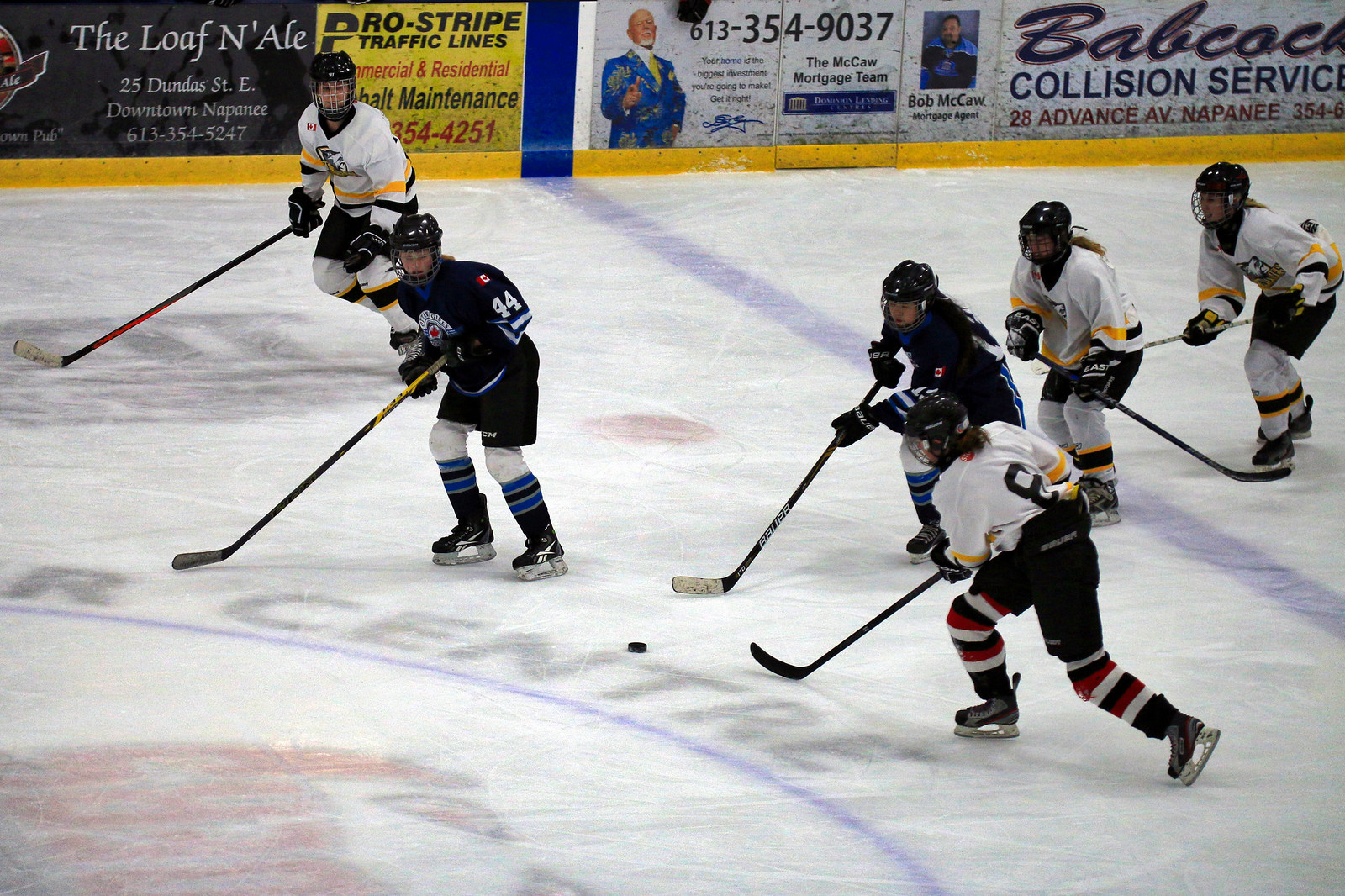The image captures an indoor youth hockey game in a stadium in Ontario. At the center-left, six hockey players focus intently on a puck. On the right, four players in distinct uniforms — three in white, yellow, and black jerseys and one in predominantly black with blue-striped leggings — move towards the puck. The closest player's jersey displays the number three. On the left of the puck, another player in black, numbered 44 on their arm, skates alongside a teammate in white and yellow. These young players, in full gear with pads and helmets, diligently chase the puck. The rink's boards feature various local advertisements, including "The Loaf and Ale" located at 25 Dundas Street East in downtown Napanee, "The Macaw Mortgage Team," a legal services ad for collision support, and "Pro-Stripe Traffic Lines." A prominent image of Don Cherry, known for his bright, flashy suits, embellishes the side of the rink, adding a familiar touch to the scene. This lively photograph showcases the energy and focus of a youth hockey league game.